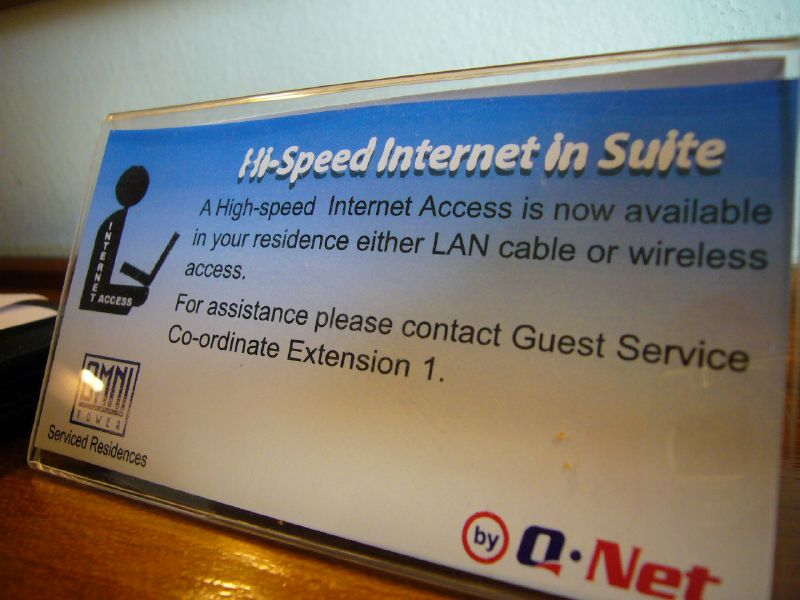The image depicts a rectangular sign, propped upright and leaning slightly back, situated on a dark brown, wood-grain table indoors. The sign features a gradient design that transitions from blue at the top to white at the bottom. This sign announces, in bold, white, bubbly lettering against a blue background at the top: "High-Speed Internet in Suite." Below, in standard black text on white, it provides the details: "High-speed internet access is now available in your residence via LAN cable or wireless access. For assistance, please contact Guest Service at Extension 1." Upon the left side of the sign, there is an outline of a person holding a laptop, paired with the text "Internet Access" in white. In the bottom left is the hotel logo, "Omni Tower Service Residences," while the bottom right exhibits the "By QNET" logo, with 'Q' in dark blue and 'NET' in red. The background reveals a white wall and some papers scattered on the table, with a light source illuminating the scene.